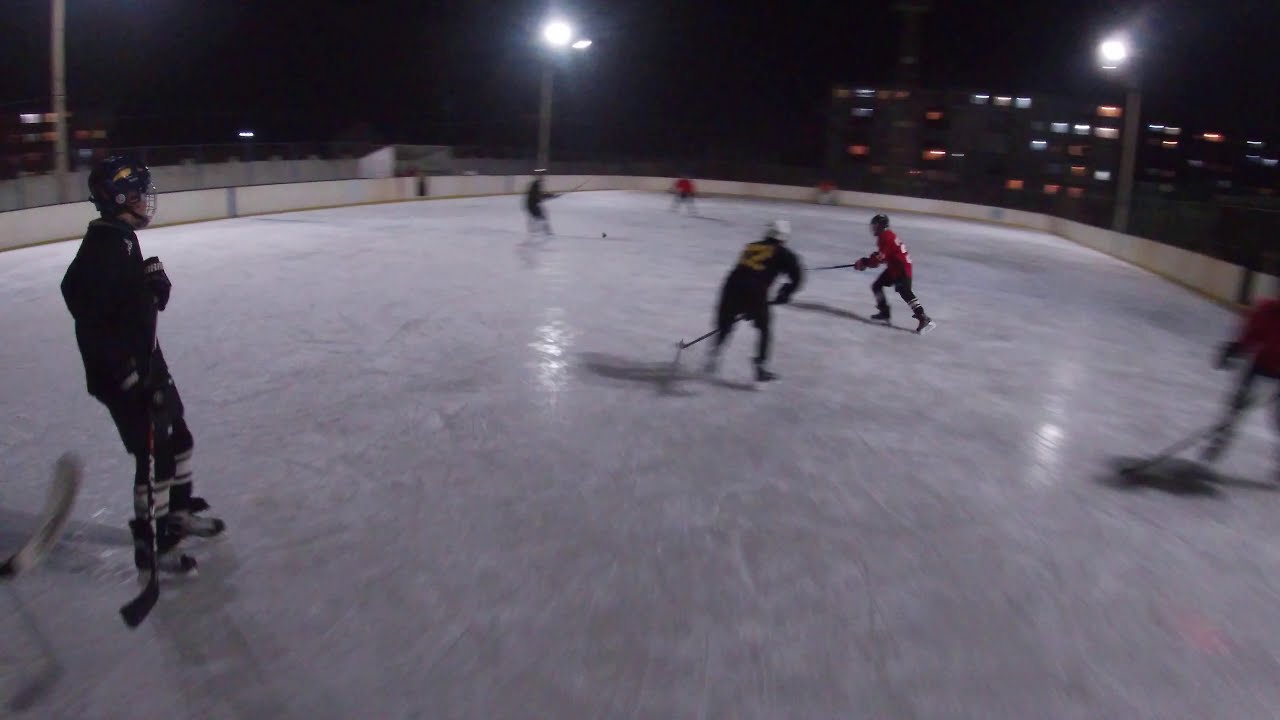This photograph captures a nighttime ice hockey match in an open stadium. The ice rink, visibly marked by extensive skate lines, is surrounded by a cream-colored barrier. The stadium lights are brightly illuminated against the black sky, highlighting the action on the ice. There are two teams, distinguished by their uniforms – one in black jerseys with black bottoms and the other in red jerseys with black bottoms. Approximately six to seven players, some reaching for the puck, are clearly immersed in the game, wearing helmets and wielding hockey sticks. The movement of the players introduces a slight blur to the image, emphasizing the game's intensity. Beyond the rink, several lit-up buildings can be seen, enhancing the ambiance of the outdoor setting.